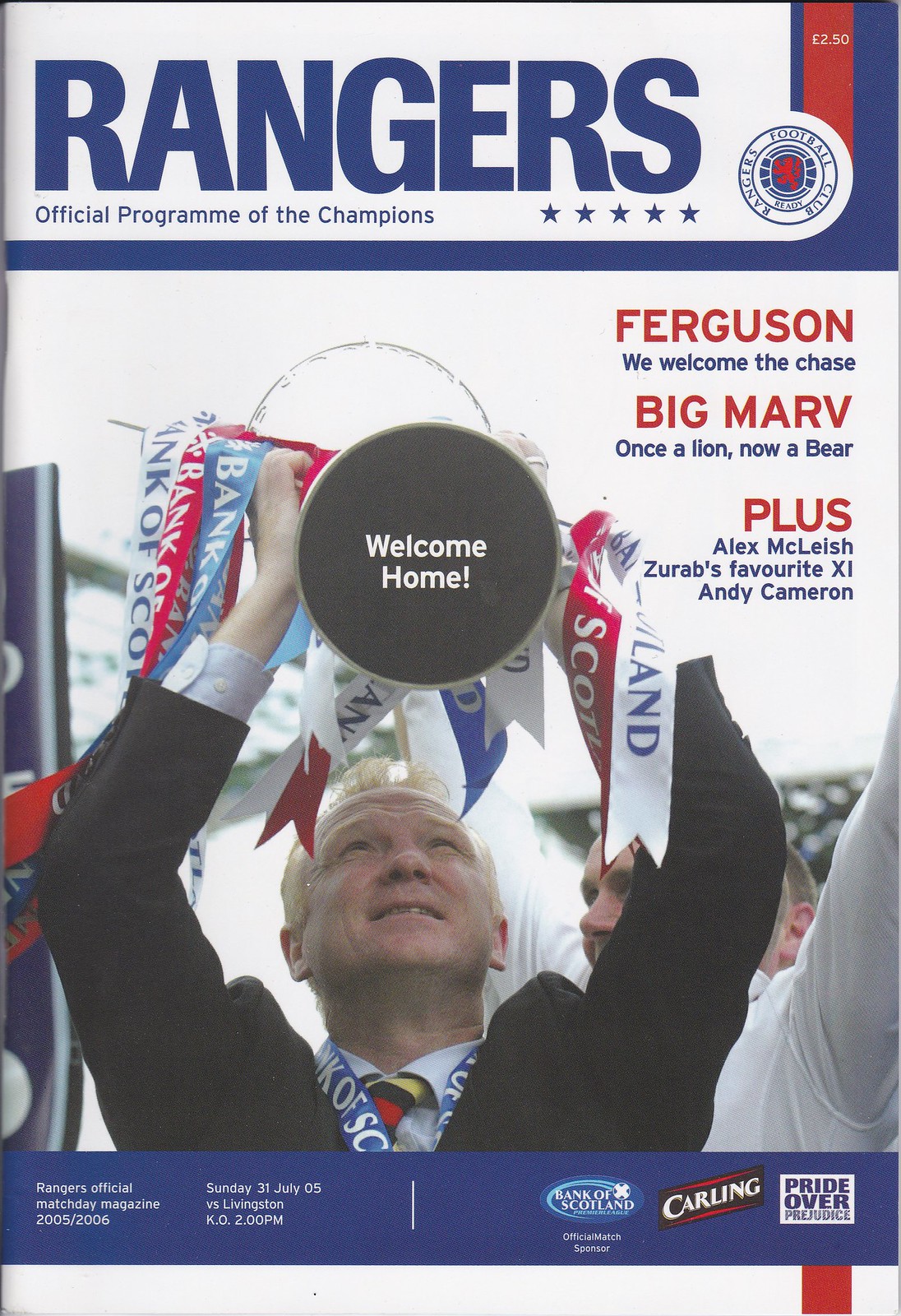The image depicts the full-color cover of an official program from a sporting event, likely a hockey championship, prominently featuring the text "Rangers Official Program of Champions" and "Welcome Home." The team's logo is positioned at the very top. Central to the cover is an older, bald gentleman dressed in a black suit, a white shirt, and a colorful tie. He is standing indoors, possibly on a hockey rink, and joyously holding a trophy high over his head, adorned with ribbons cascading down. Surrounding the gentleman, various inscriptions can be seen, including "Ferguson we welcome the chase," "Big Marv, once a lion now a bear," "Alex McGlay," "Zoo Rob's favorite," and "Andy Cameron." The overall color scheme of the program is red, white, and blue, adding to the celebratory and patriotic feel of the event.